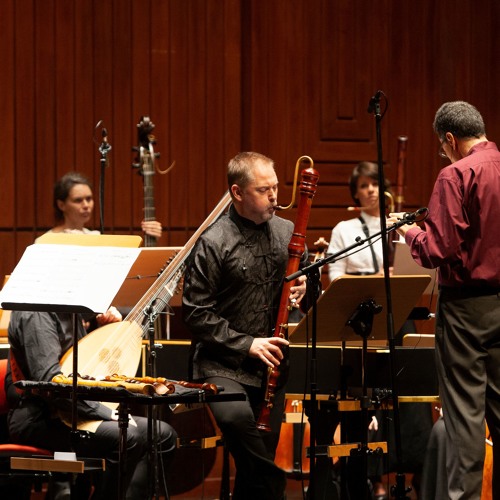The image depicts a classical music ensemble, potentially during a rehearsal or performance, set against an elaborate wooden-paneled backdrop that exudes an air of sophistication. On the right, a conductor, clad in gray slacks and a long-sleeved red shirt with glasses, is poised on a platform, guiding the musicians. To his left, a musician is performing a solo on a distinctive long wooden wind instrument, which arches up to meet his mouth—possibly a bassoon. Adjacent to him, another seated musician is playing a stringed instrument characterized by a long neck and an oval body, resembling an oversized lute or mandolin. In the background, two women stand with their instruments; one holds hers without playing, while the other cradles a large cello. This meticulously controlled environment suggests a professional setting, possibly a concert hall, underscored by the presence of music stands with sheet music.